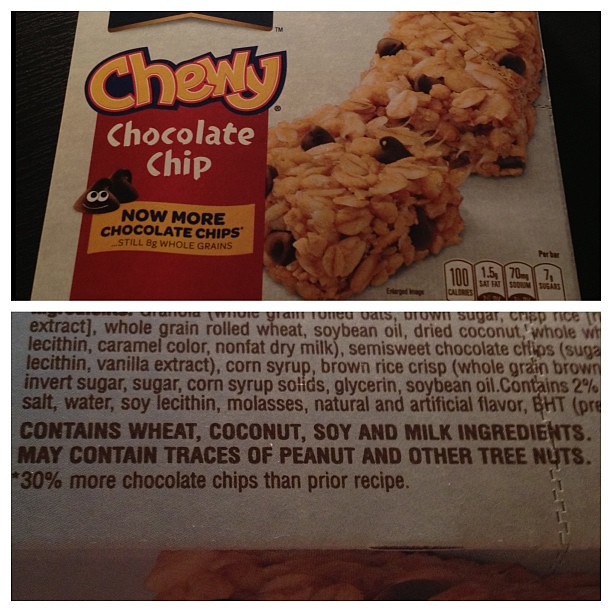The image showcases a close-up view of a granola snack package from Quaker Oats, specifically their Chewy Chocolate Chip variety. The composition includes two pictures, both rectangular and oriented horizontally. The top picture prominently displays the product packaging, featuring a granola bar integrated with chocolate chips, shown broken in half. The box is labeled "Chewy Chocolate Chip" with an eye-catching vertical red banner that reads "Now More Chocolate Chips." There is also a playful image of a chocolate chip with eyes and a smile, accompanied by text stating "still eight whole grains," and some nutritional information on the bottom right. The bottom picture is a zoomed-in snapshot focusing on the ingredients list, although the top portion is missing. It highlights key ingredient information, including a bold statement: "Contains sweet coconut, soy, and milk ingredients. May contain traces of peanuts and other tree nuts," and emphasizes "30% more chocolate chips than prior recipe."